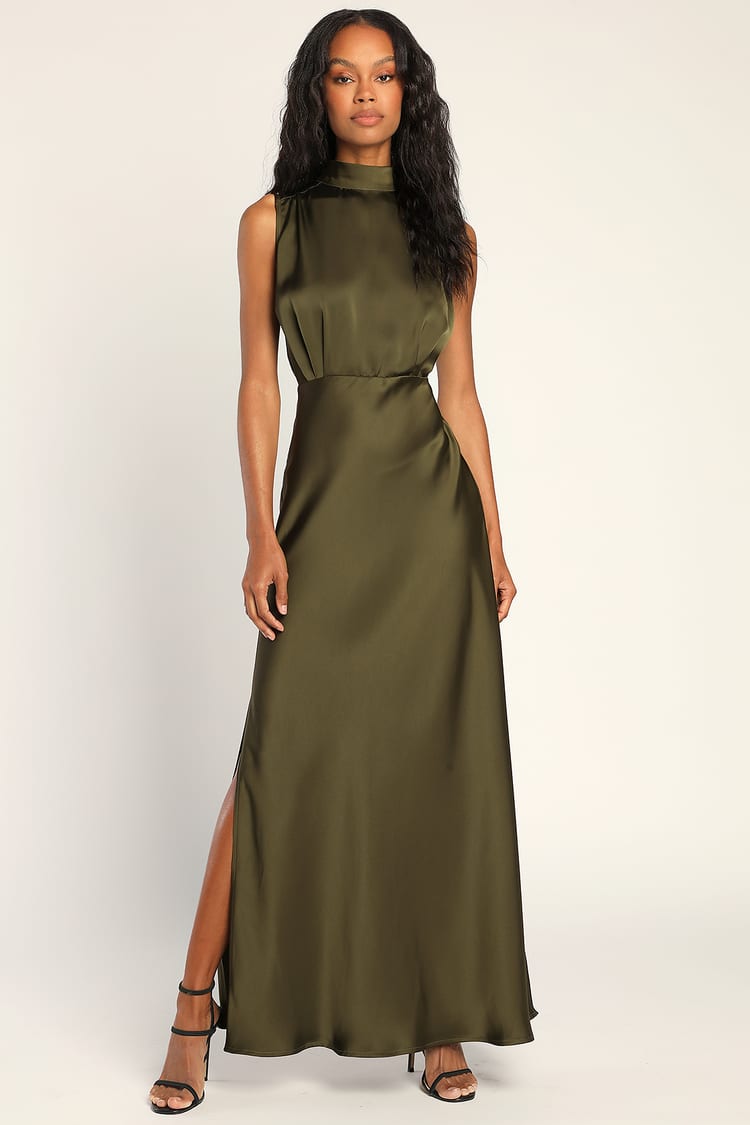In this photograph, a young, light-skinned model stands confidently in front of a white backdrop, casting a slight shadow. Her shoulder-length black hair frames her face, which carries a serious yet slightly smiling expression. She is wearing a floor-length, olive green dress made of shiny, satiny fabric that is sheer and cinched at the waist. The dress features a mock turtleneck and is sleeveless, with a small slit at the bottom reaching up to almost the knee, revealing her right leg. Her hands are relaxed at her sides, and she completes her look with black, strappy high-heeled sandals. The photo captures the model from the front, showcasing her poised and elegant stance.